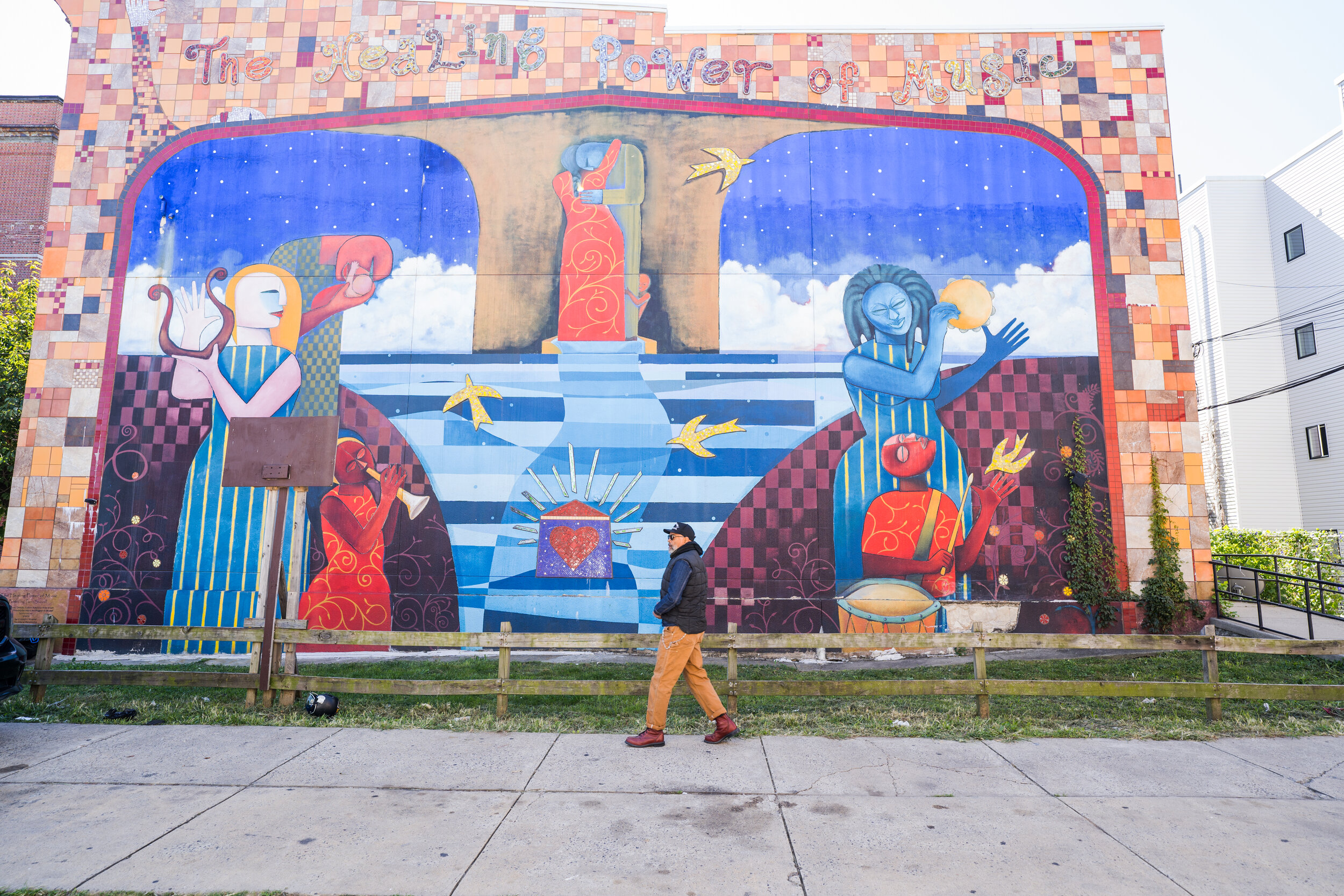A vibrant mural painted on the side of an outdoor building depicts a surrealistic scene filled with musical motifs. The background is a vivid mix of colors, including blues, reds, yellows, and oranges, creating a dynamic and whimsical atmosphere. The mural unfolds from left to right, starting with a blonde woman with fair skin wearing a long blue dress adorned with yellow vertical stripes. She seems to be intently playing a harp. Beside her is a black woman in a red dress with yellow floral patterns, passionately blowing into a horn.

Moving further right, the central part of the mural features an enigmatic figurine decorated with spikes, surrounded by various yellow birds depicted as abstract designs. The scene's continuity introduces another character, a blue-skinned lady with matching blue hair, dressed similarly in a blue outfit with yellow stripes. She is holding a yellow tambourine against a rich red and burgundy background. 

In front of this blue lady stands another figure with red attire and a red hat, facing away with an outstretched arm that seems to hold a yellow bird. This entire feast for the eyes is set against a painted sky of blue with floating white clouds. At the summit of the mural, indistinct writing reads something akin to "the real power of music," though the exact words are hard to decipher due to overexposure.

In front of this elaborate mural, a heavyset older man with white skin walks down a clean concrete sidewalk. He wears yellow pants, a blue jacket, and a black hat, oblivious to the colorful wall art behind him. The mural is bordered by a wooden fence, although weathered and moldy, diligently preserving the scenery. The surroundings are neat, with no trash in sight, and flanked by buildings in white and red, enhancing the mural's wide-ranging impact. This mural invokes a sense of a musical heaven, with characters poised in what appears to be a temple under a starlit sky, creating an enchanting and lively tableau.